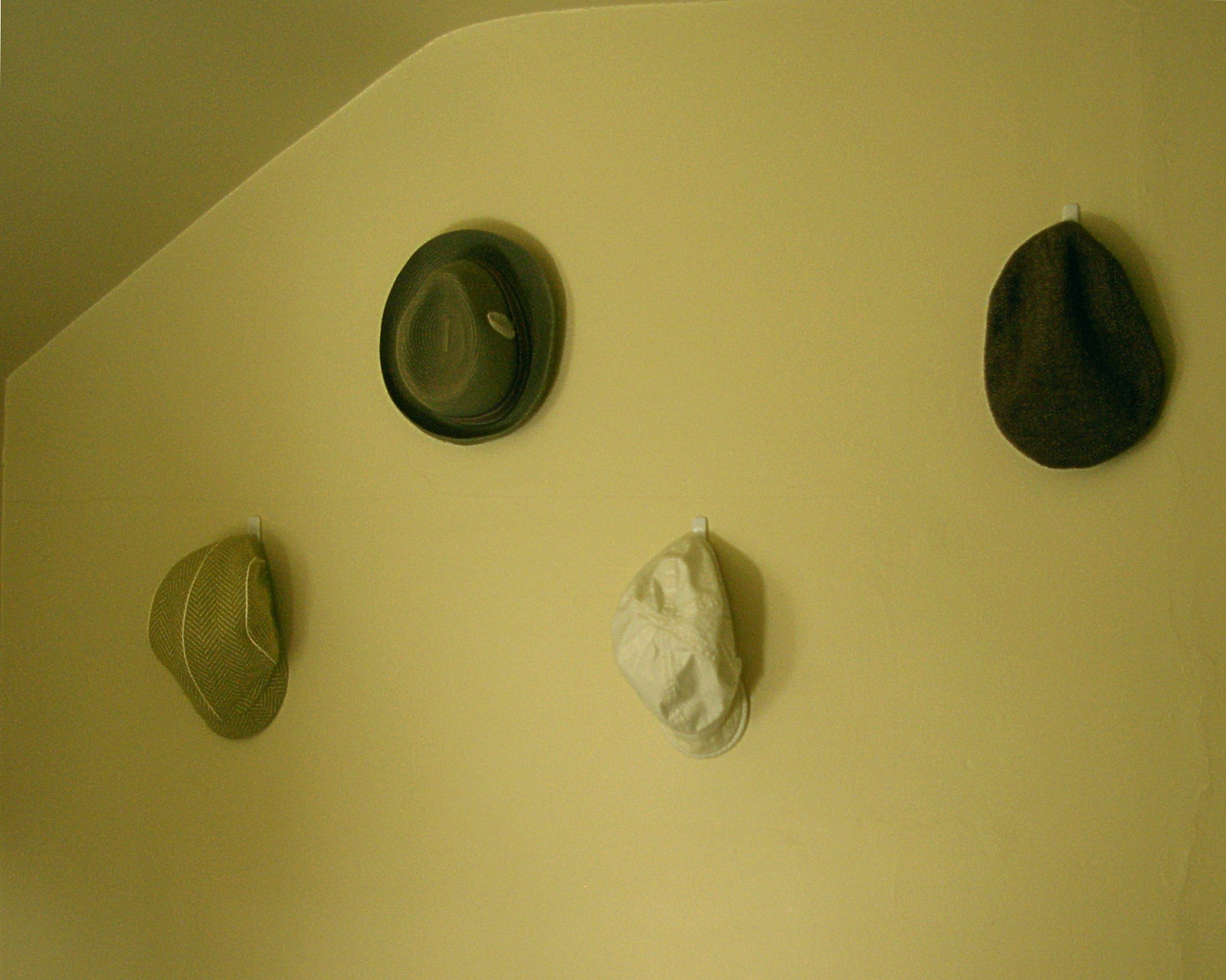The image captures a photorealistic scene featuring a yellow-tinted wall adorned with four hats, all mounted on white pegs. The wall's color, a faded mustard yellow, possibly lightened by a greenish hue, extends across most of the image, with the top left corner transitioning into a darker shade. On the left side of the wall, a brown newsboy cap with yellow stripes hangs, its texture slightly wrinkled. Above it, slightly to the right, is a green bowler hat with a dark brown band and a lighter green accessory. Centrally positioned, a white baseball cap sits below a dark gray trilby hat adorned with a black sash or band. On the far right, a dark gray beret is mounted. The arrangement and lighting suggest the setting may be a gallery or commercial space rather than a domestic interior.